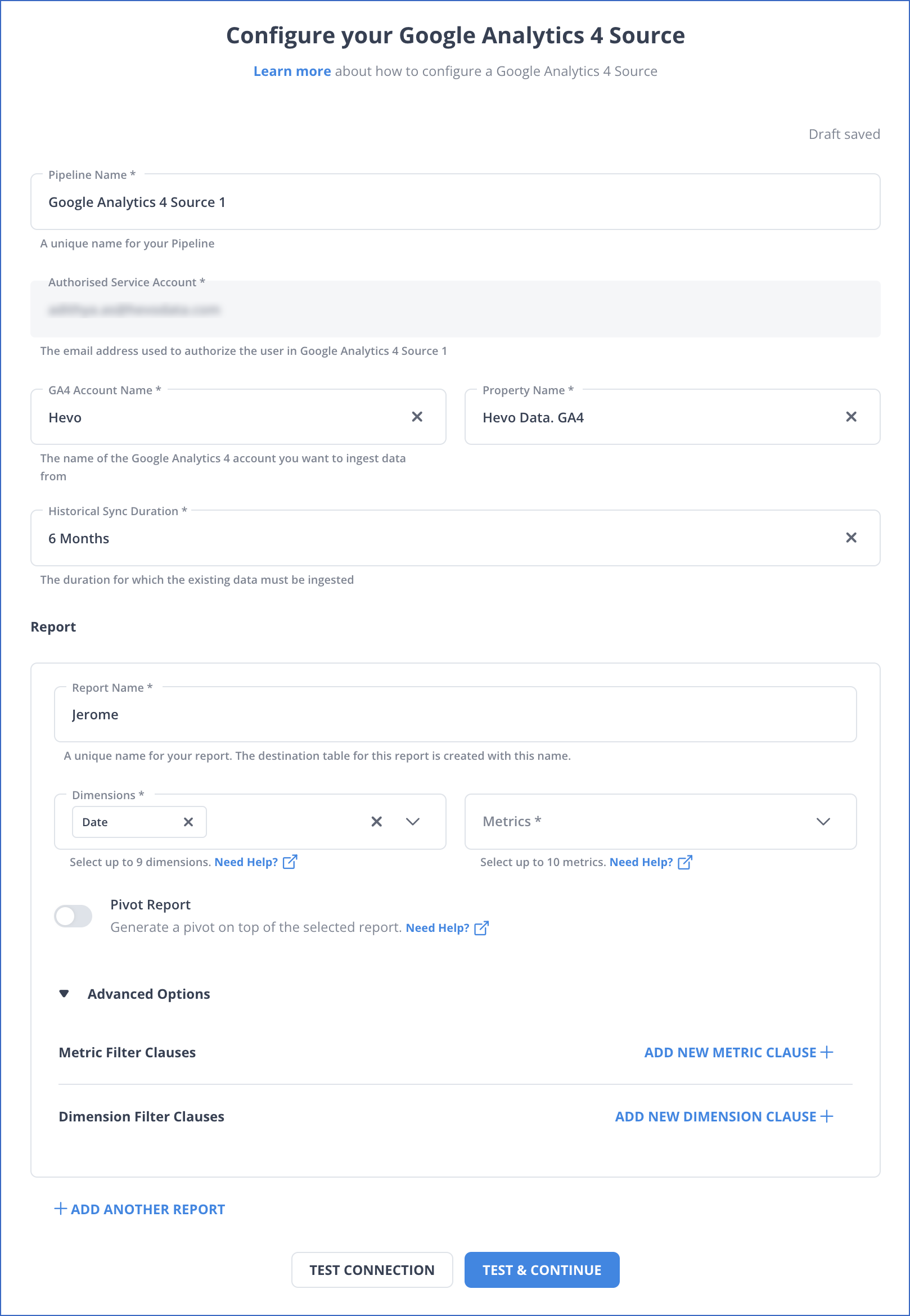**Detailed Caption:**

The image is a screenshot from a website featuring a white background with a thin, dark blue border. At the top-center of the image, there is prominent bolded text that reads "Configure Your Google Analytics 4 Source." Directly beneath this, in smaller blue lettering, is a "Learn More" link, followed by black text stating, "about how to configure a Google Analytics 4 source."

On the right side of the image, there's text indicating "Draft saved." 

On the left side of the image, there is a large rectangular bar resembling a search bar, which spans the width of the section. The bar is labeled "Pipeline Name" at the top-left corner, with bold text below it reading "Google Analytics 4 Source 1." Below the bar, outside of it, there is an annotation saying "A unique name for your pipeline."

Further down, there's a gray-bordered, long rectangular area with blurred-out words. Above these blurred words, a heading reads "Authorized Service Account," and directly beneath it, there is a description stating "The email address used to authorize the user in Google Analytics."

Below this section are two search bars labeled "Account Name" and "Property Name." Additional information follows below these search bars, leading to another search bar labeled "Historical Sync Duration," with descriptive text beneath it.

Continuing down, there is bold text that says "Report," followed by a large square labeled "Report Name" accompanied by a search bar. Adjacent to this are date dimension fields, and on the right side, there is a search bar for metrics.

Below these sections, there are multiple tabs available for assistance. Under this, there's a toggle switch on the left that is currently set to off, with text next to it reading "Pivot Report."

Directly beneath, there is an informational line followed by text in black that says "Advanced Options," with a dropdown tab to its left. Lower down, there are sections titled "Metric Filter Clauses" and "Dimension Filter Clauses," each with "Add New Metric Clause" and "Add New Dimension Clause" options featuring blue plus signs.

At the bottom-left of the image, there's a plus sign labeled "Add Another Report" next to a white pop-up tab that reads "Test Connection" in black, and a blue tab stating "Test and Continue" in white.